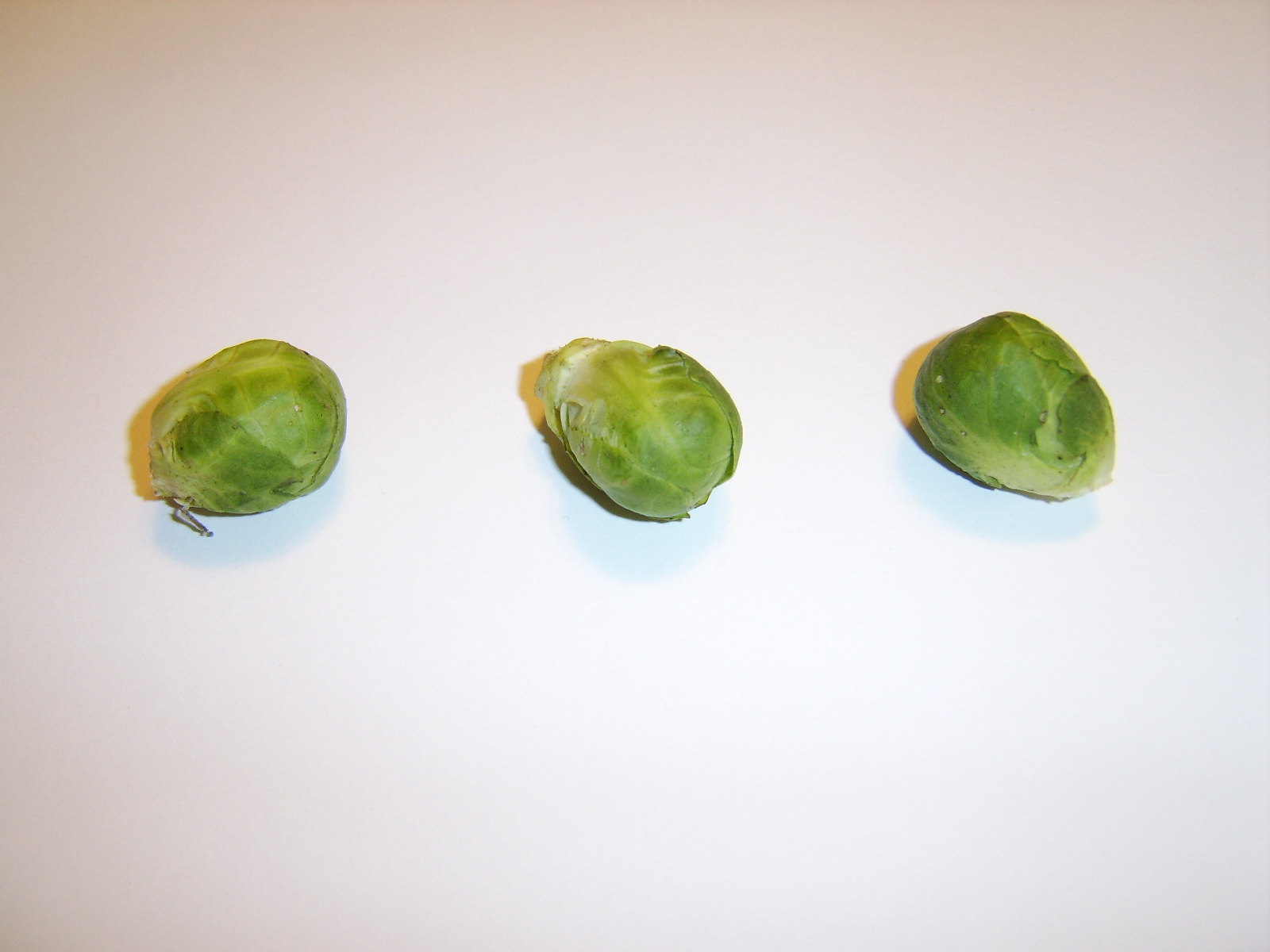This photograph captures three fresh Brussels sprouts, meticulously arranged in a horizontal row across an undefined white surface, possibly a countertop or a piece of paper. Each Brussels sprout, resembling tightly wound miniature cabbages, is uniform in size yet varies slightly in orientation. The leftmost sprout points towards the upper right with a visible dried leaf at its bottom, the middle one faces the upper left with its cut base prominent, and the rightmost one directs its base downwards and to the right, displaying faint brown marks.

The vibrant green hues of the Brussels sprouts exhibit a gradient, transitioning from white at the base to a darker green at the top, highlighting their fresh, uncooked state. Illuminated by a bright light source from the top right, the sprouts cast sharp, bluish-green shadows diagonally to the upper left, with an additional softer shadow falling beneath them. The background, although predominantly white, hints at a subtle, pinkish tinge that fades towards the center, possibly due to the lighting conditions. The overall image, taken from a top-down perspective, emphasizes the intricate textures and natural details of the Brussels sprouts against their stark, minimalist setting.